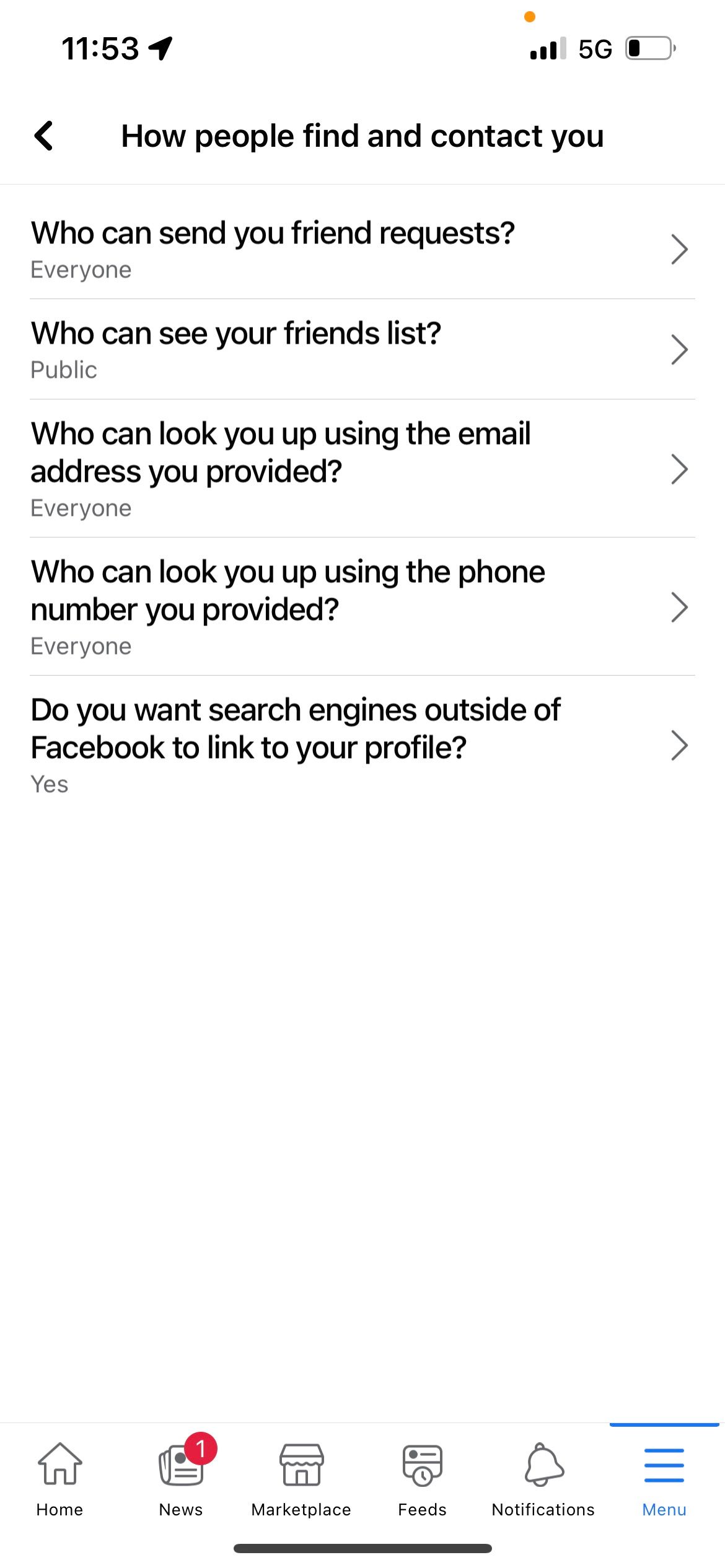**Caption:**

This is a detailed screenshot of a cell phone image taken at 11:53 (either AM or PM). The device shows the location services enabled, with the upper-right section indicating that the phone has 75% network reception on a 5G network and a battery level at about 25%. 

Displayed prominently on the screen, within a "How People Find and Contact You" section, there is a back arrow to the left of this heading. The options listed underneath include:
- "Who can send you friend requests?" which is set to "Everyone" and features a right arrow to indicate a drop-down menu.
- "Who can see your friend list?" set to "Public," again with a right arrow.
- "Who can look you up using the email address you provided?" set to "Everyone."
- "Who can look you up using the phone number you provided?" set to "Everyone."
- "Do you want search engines outside of Facebook to link to your profile?" with the answer marked as "Yes."

At the bottom of the screenshot, the navigation bar displays options for "Home," "News," "Marketplace," "Feeds," and "Notifications" along with a menu icon represented by three horizontal lines.